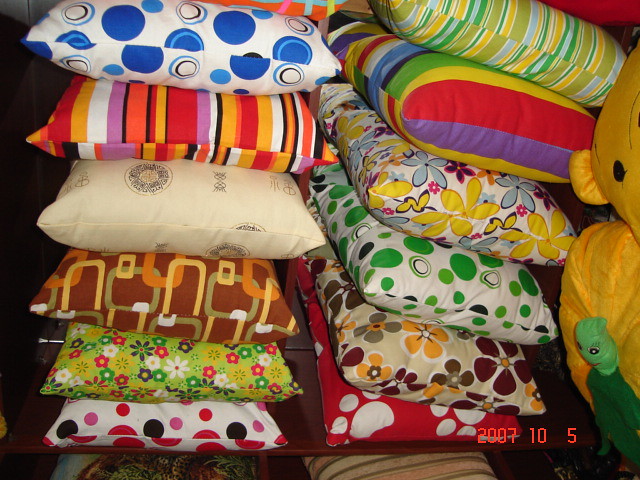The photograph, dated "2007-10-5" in pixelated red font on the bottom right, features a close-up display of two stacked columns of ten colorful couch pillows each, arranged on a dark brown wooden shelf. The left column showcases pillows with diverse designs: a white pillow with blue circles, a pinstripe pattern in white, yellow, purple, orange, and red, an ivory pillow with abstract details, a dark warm brown pillow with orange, yellow, and green rectangles, a green pillow adorned with yellow, red, white, and green flowers, a white pillow with red, pink, and black polka dots, and several others in varied colors and patterns. The right column displays an equally varied collection with designs, including a striped mix of green, blue, yellow, and other bold colors, large floral prints, and geometric patterns. Adjacent to the pillow stacks on the right side, a plush yellow bear and a smaller green creature, possibly a turtle or an alien, are also visible, adding whimsical elements to the scene.